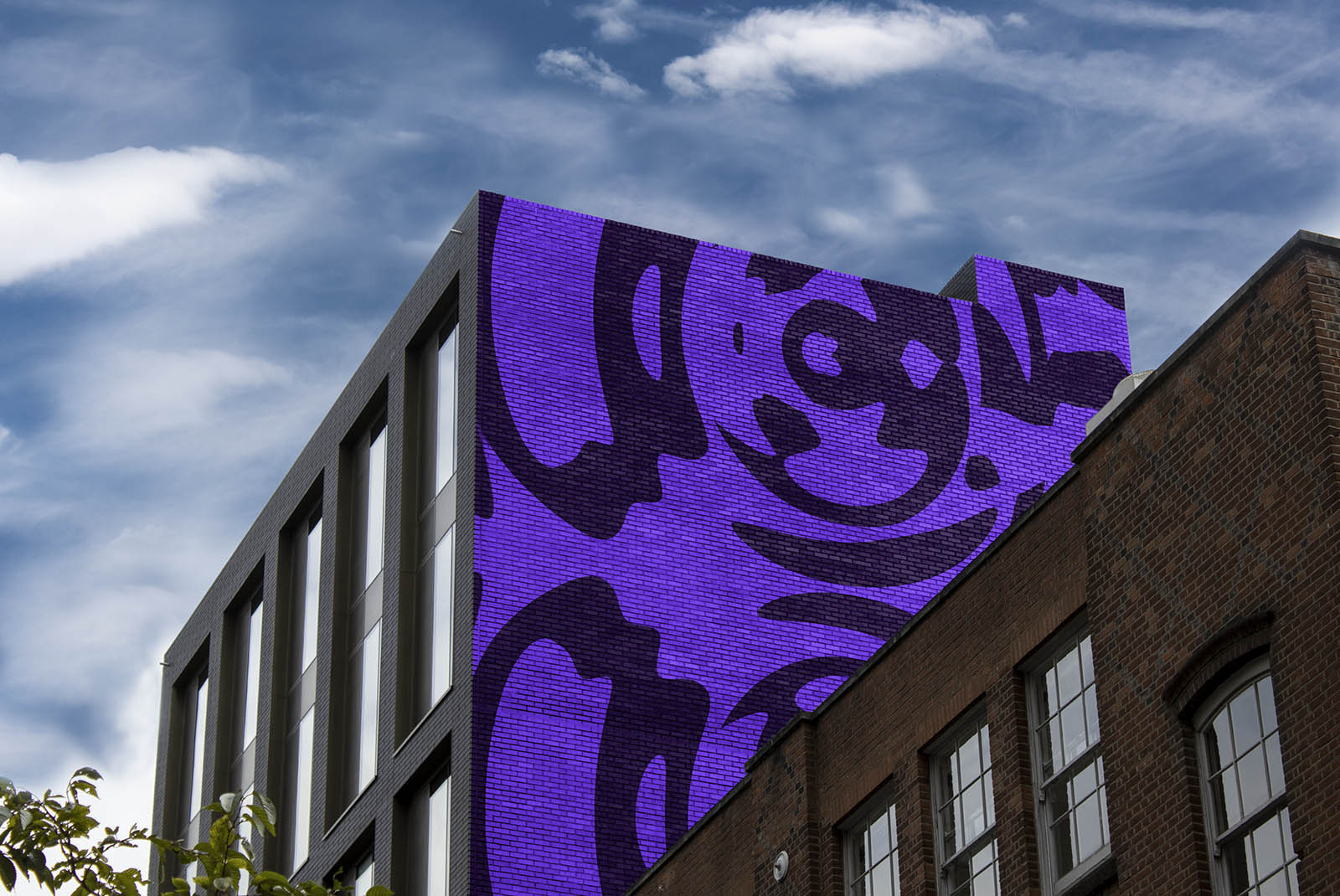The image depicts a vibrant cityscape with a striking mural on the side of a dark brick building. The building features large glass windows on its front, reflecting a brilliant blue sky dotted with both white and dark wispy clouds, and a possible chemtrail in the top right corner. Rising into the sky, the mural on the building’s right side is an abstract composition of geometric swirls in deep purple and black, contrasting with the building's darker tones. The building next to it, a shorter structure made of red and brown bricks, also has numerous windows and a white roof vent. In the bottom left corner of the image, part of a green-leafed tree is visible. The photograph is taken from a ground-up perspective, capturing the grandeur and artistic flair of the tall building against the expansive sky.